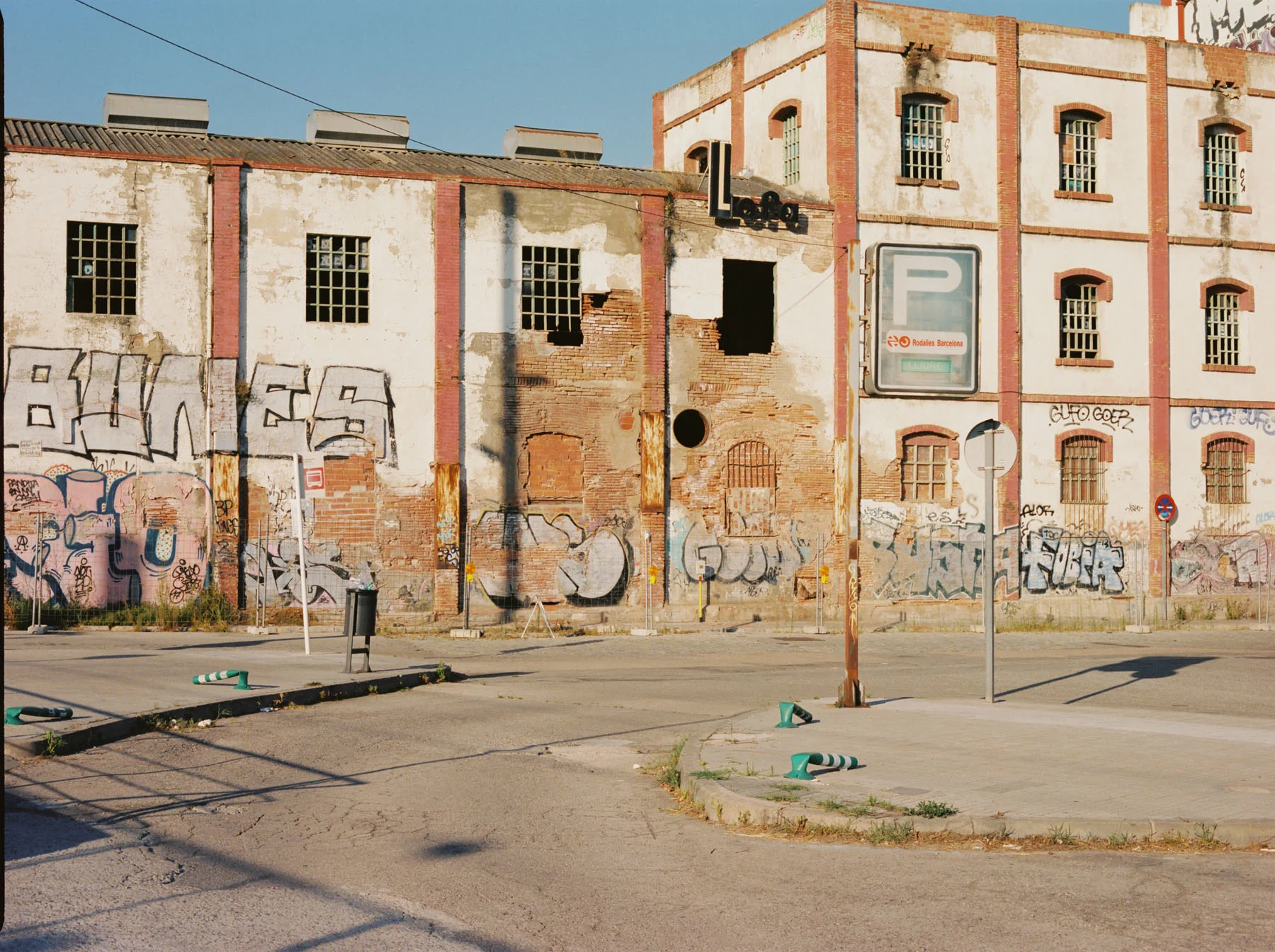The image captures a dilapidated, seemingly abandoned urban area. In the foreground, cracks crisscross the pavement, with grass and dead weeds pushing through, indicative of long-term neglect. The cement space is sporadically marked by signs. The structure in the background is substantial and divided into seven or eight sections, with the segments on the left being noticeably shorter than those on the right. The left sections feature three large grated windows amidst exposed, deteriorated brick where the paint has peeled away, and are heavily adorned with graffiti and boarded-up windows. The building's grimy exterior is predominantly off-white, accented by faint industrial red pillars. The right sections stand taller, organized in a grid of three windows across by three down, equally marred by broken glass, graffiti, and signs of decay. The entire area, beneath a clear sky, evokes a strong sense of abandonment, with a stark contrast between the overgrown vegetation and the derelict, graffiti-laden architecture.